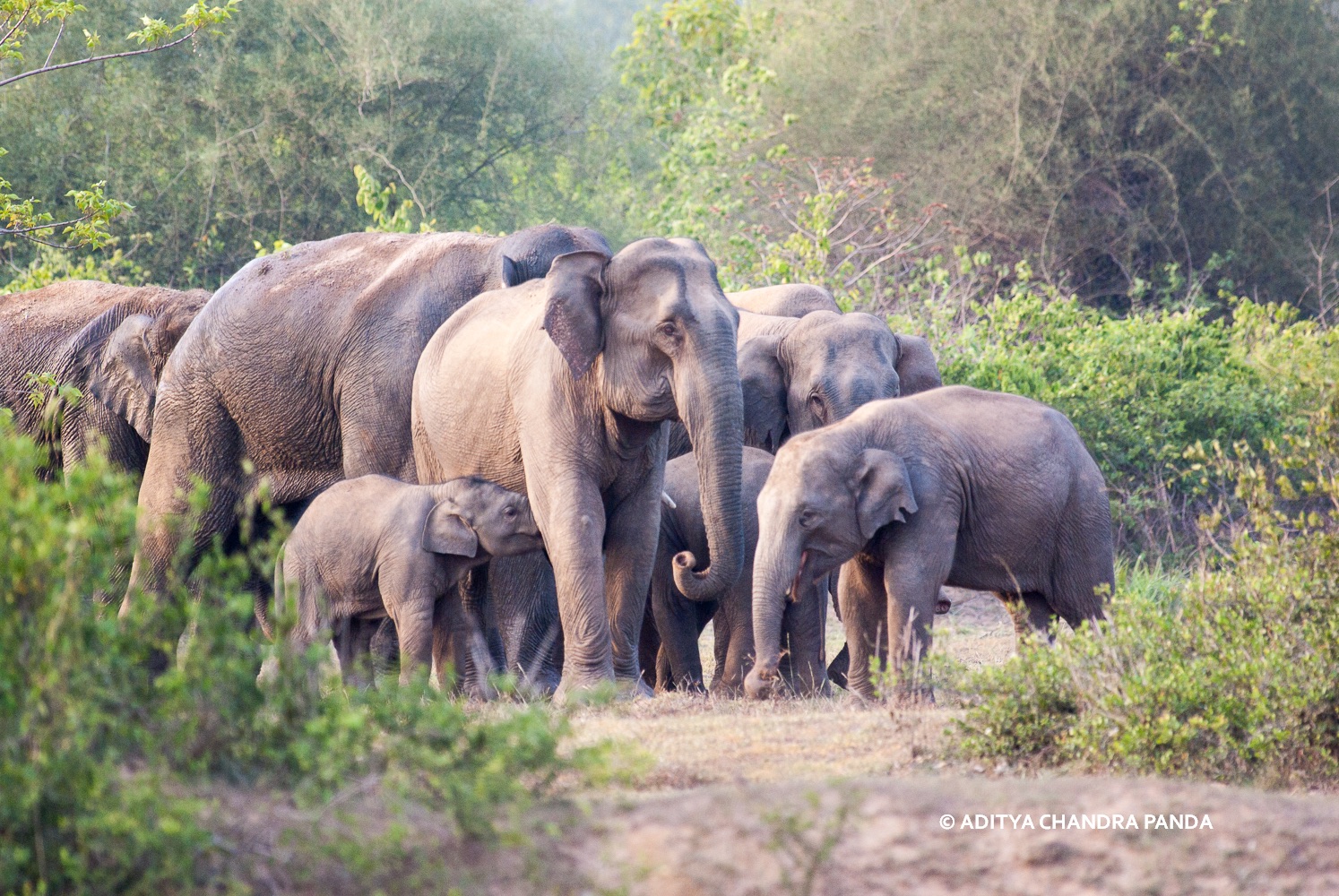The full-color photograph, which is horizontal and rectangular in shape, captures a closely grouped herd of elephants in a lush, green clearing. The central figure is a large mother elephant oriented to the right, with her baby nestled underneath, its head and trunk tucked beneath her front right leg. In total, there are five adult elephants, one baby, and two juveniles, all varying shades of gray. One juvenile, eyes closed, faces to the left. Lush greenery with tall shrubs and trees surrounds the herd, while a brown dirt path extends toward the foreground. The overall palette contrasts the gray of the elephants against the vibrant green backdrop. At the bottom right, white text reads, "At Aditya Chandra Panda."